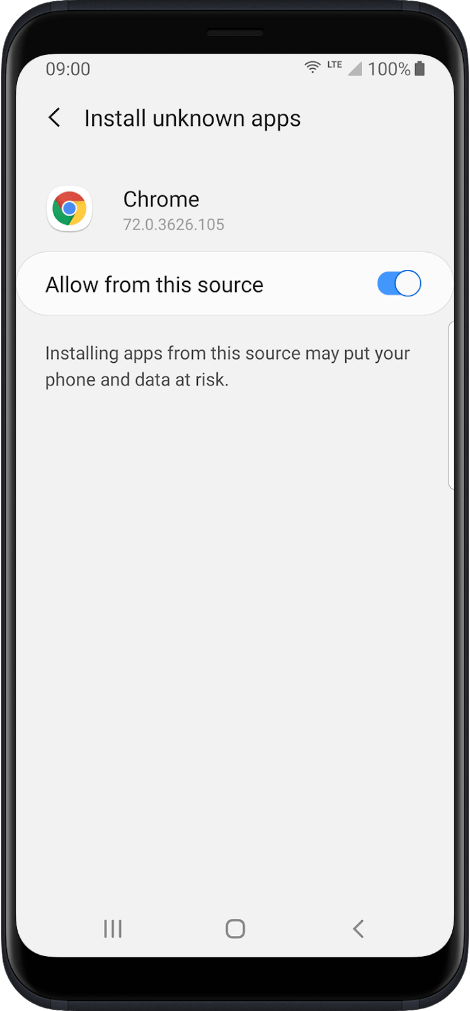The image depicts a black smartphone displaying a screen with a predominantly white background and a slight gray tint. The status bar at the top of the screen indicates the time as 9:00, with the battery at full charge (100%) and a Wi-Fi connection active. Central to the image is a heading reading "Install unknown apps," accompanied by a left-facing arrow icon to its left. Below this, the Google Chrome icon is prominently displayed, characterized by a white circle with a multicolored circle inside and a blue center, alongside the label "Chrome." Further down, a long oval white bar contains the text "Allow from this source," with a blue toggle switch positioned on the right side, indicating that the option is enabled. At the bottom, a smaller text warning cautions, "Installing apps from this source may put your phone and data at risk." The overall context suggests that the user is in the process of enabling the installation of an app from an unknown source, with the device providing a security warning about potential risks.